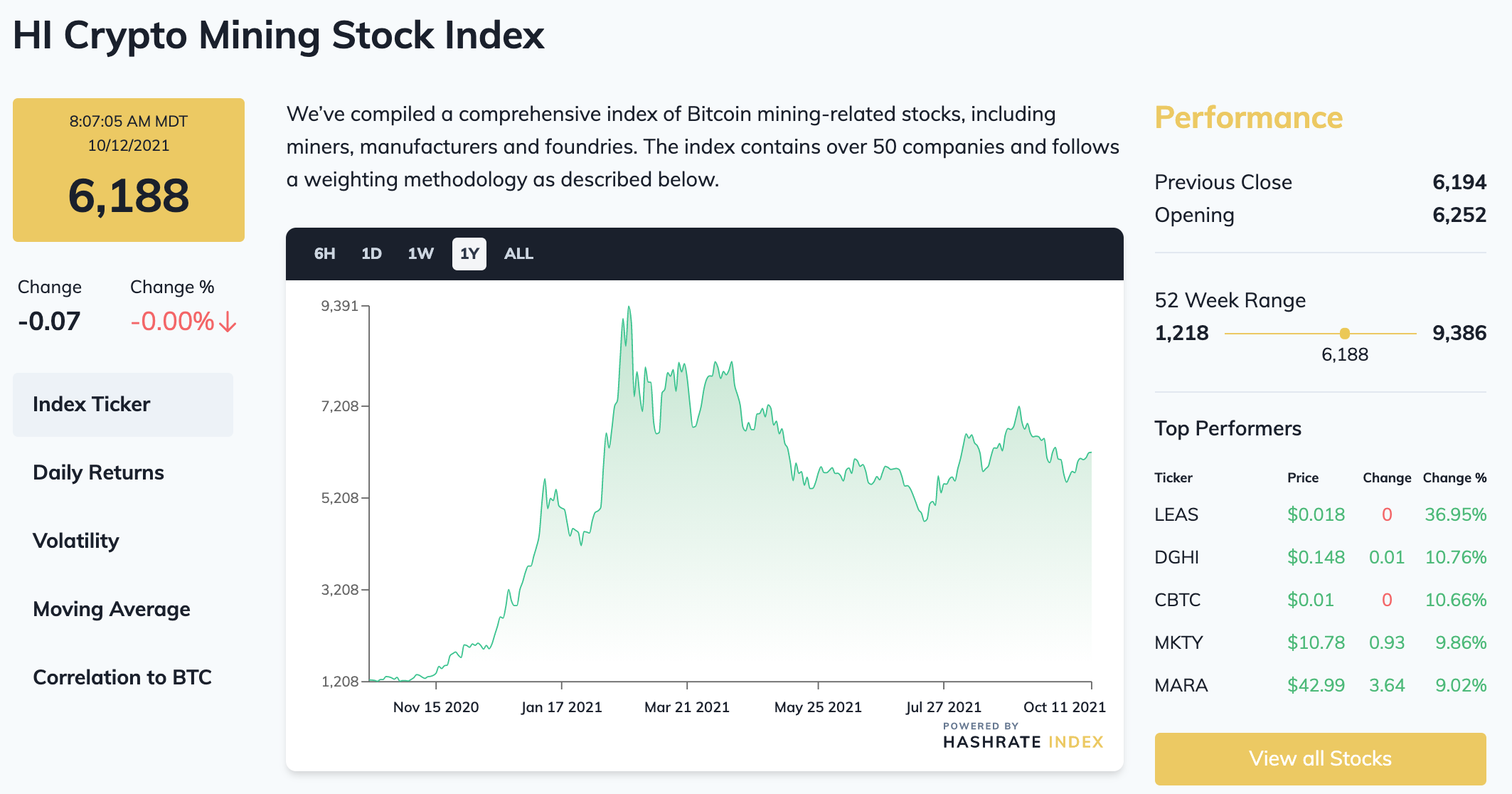**Detailed Caption:**

This image is a screenshot of a financial website dedicated to tracking the Crypto Mining Stock Index. In the top left corner, the header "HI Crypto Mining Stock Index" is prominently displayed. Directly underneath, the current date and time are indicated: 8:07:05 AM MDT on October 12, 2021. The index value is shown as 6,188, set against a yellow rectangle background. Below the index value, the "Change" is noted as -0.07, accompanied by a red downward arrow. The "Change Percentage" is also specified as -0.00%.

Further down, various financial metrics are listed, including "Index Ticker," "Daily Returns," "Volatility," "Moving Average," and "Correlation to BTC." To the right of these metrics, a detailed line graph is displayed, illustrating the index's performance over time. The accompanying text mentions that this index comprises over 50 companies involved in BTC mining, including miners, manufacturers, and foundries, and follows a specific weighting methodology.

The graph offers several time frame options for viewing, such as 6 hours, 1 day, 1 week, 1 year, and all-time, with the current view set to "1 year." On the right side of the screen, additional performance metrics are presented: "Pre-Closed" value of 6,194 and "Opening" value of 6,252. A "2 Week Range" is also displayed, showing a range from 1,218 to 9,386.